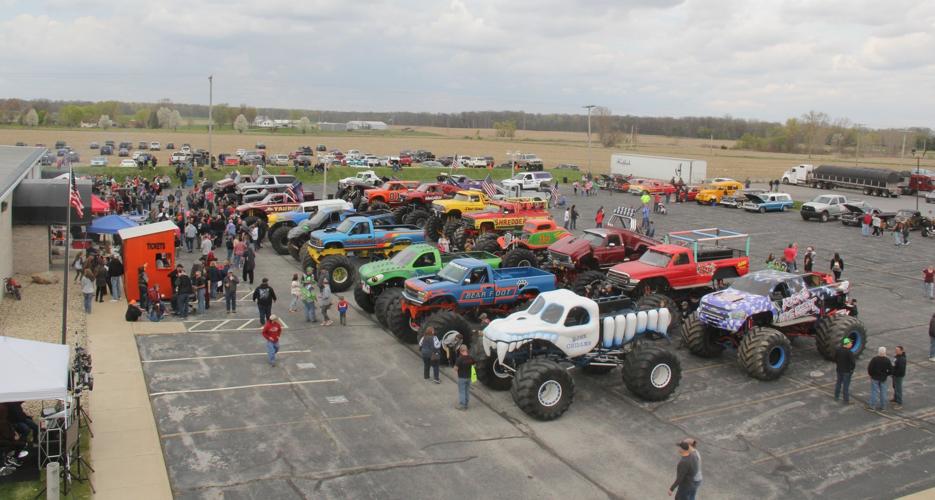The image depicts a large outdoor parking lot filled with an array of vividly painted monster trucks, featuring enormous, oversized wheels. The trucks' bodies come in a variety of colors, including white, blue, bright green, red, and purple, with intricate and creative designs such as a dragon skull, an alligator, and red teeth. They are neatly lined up in rows within designated parking spaces. The scene is lively with numerous people, including adults and children, walking around, enjoying what appears to be a monster truck show or race event. The sky above is predominantly cloudy, with patches of blue occasionally peeking through. In the background, there are fields of green and brown grass, a few buildings on the left side, some with American flags, and a little red booth along with a white-roofed tent. Beyond this, one can see hills, trees, houses, and additional vehicles, contributing to the overall bustling and festive atmosphere of the event. The photo is taken from a slightly elevated, top view angle, capturing the expansive scene in a horizontal frame.